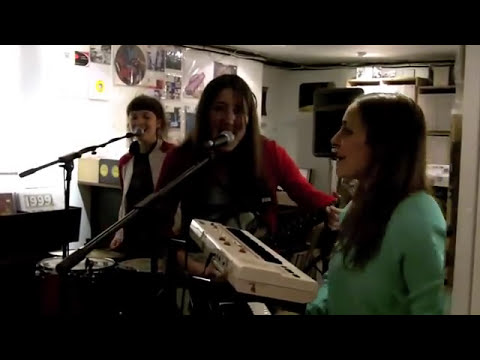The photograph, seemingly an older home or YouTube video from 1999, depicts a lively scene of three women in a small recording studio or basement. The image is framed with black bars at the top and bottom, giving it a slightly pixelated, low-resolution quality. The room is predominantly white with a white ceiling and black molding, adorned with eclectic artwork and large speakers in the background. The light source comes from the left.

On the far right, closest to the camera, a woman with long brown hair is immersed in playing a double-layered keyboard—white on top and black on the bottom—while wearing a green sweater. In the middle, another woman with brown hair, worn down, sings passionately into a microphone. She is dressed in a red cardigan over a black shirt. The third woman, on the left, sports a white jacket with red sleeves. She has brown hair with bangs and appears to be enthusiastically singing into a microphone, possibly with drumsticks in her hands and a drum set in front of her.

The trio, who look like they are thoroughly enjoying their performances, bring a sense of fun and camaraderie to the space, enhancing the dynamic and energetic ambiance of the image.